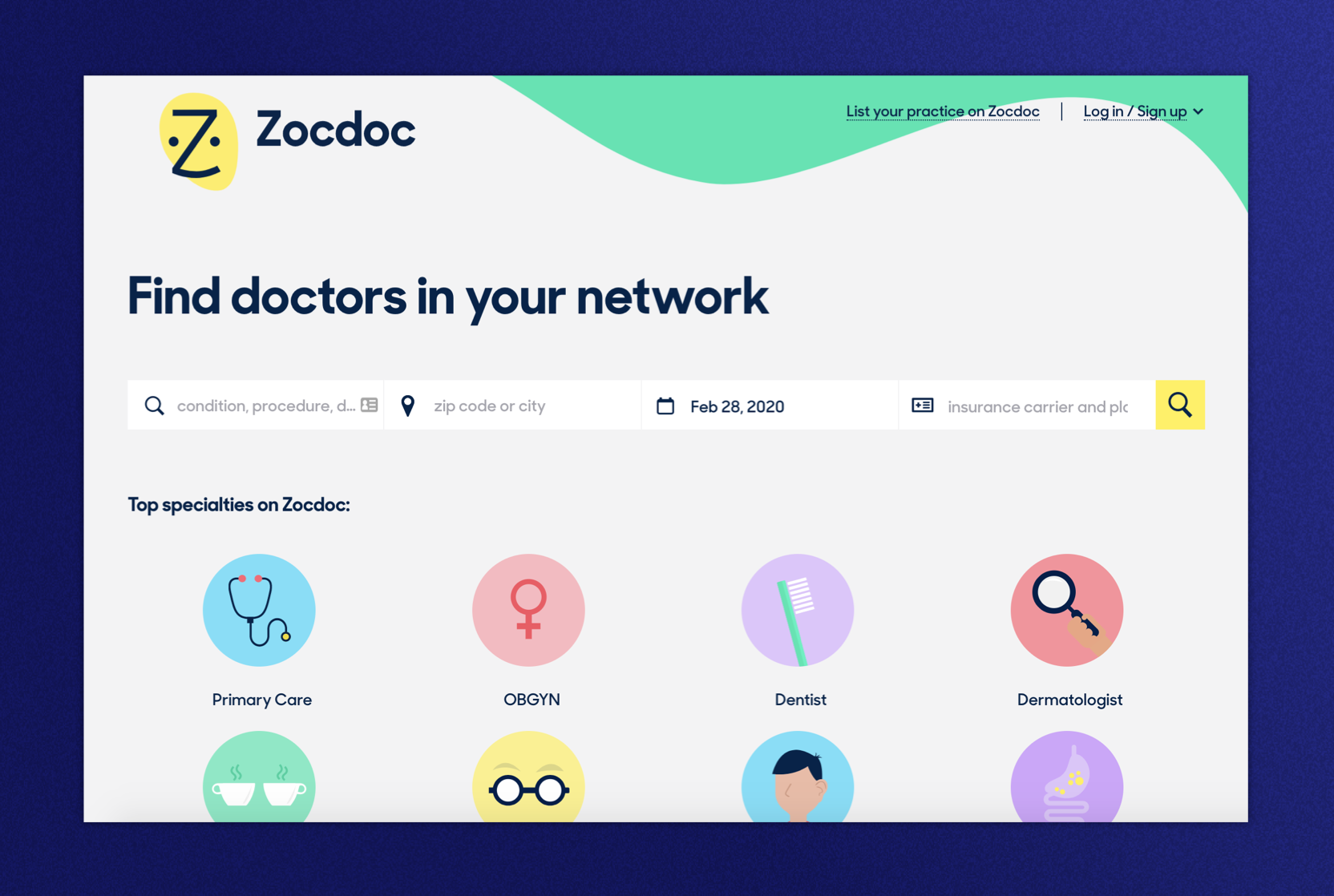The image depicts a tablet screen displaying the ZocDoc application. The interface features a prominent blue border approximately an inch thick, encasing the entire screen. At the center is a visually appealing logo on a yellow background resembling a thumbprint. The logo includes a blue 'Z' flanked by two dots, one on the left and one on the right, creating an impression of a face with an eye and a nose, giving it a cute appearance. The background of the screen is primarily gray with a noticeable green swirl in the top right-hand corner.

At the top of the screen, the text reads, "List your practice on ZocDoc," which is a clickable link. Adjacent to it, there's a "Log In/Sign Up" option with a drop-down menu. Below this header, the bold text "Find Doctors in Your Network" is prominently displayed. 

The interface includes a search bar labeled "Condition/Procedure" accompanied by an icon of a magnifying glass and a symbol of a person with three lines next to it. Adjacent to it is another search box for entering a zip code or city, marked by a pin icon. To the right, there's a calendar icon displaying the date "February 28th, 2020." Further to the right, a text box labeled "Insurance Carrier and PLA" can be partially seen, along with an icon of a card with a plus sign.

Below the search section, a yellow box with a blue magnifying glass icon is present. Underneath this, the category "Top Specialties on ZocDoc" is listed, featuring symbols for various medical specialties such as:

- Primary Care: Represented by a stethoscope on a blue circle background.
- OBGYN: Depicted by a woman symbol inside a pink circle.
- Dentist: Shown as a green toothbrush inside a purple circle.
- Dermatologist: Illustrated by a hand holding a magnifying glass inside a pink circle.

The screen also shows partial images of other items such as two coffee cups, a pair of eyeglasses, a person icon, and a cartoon drawing of a digestive tract. However, the text describing these icons is cut off and not fully visible on the screen.